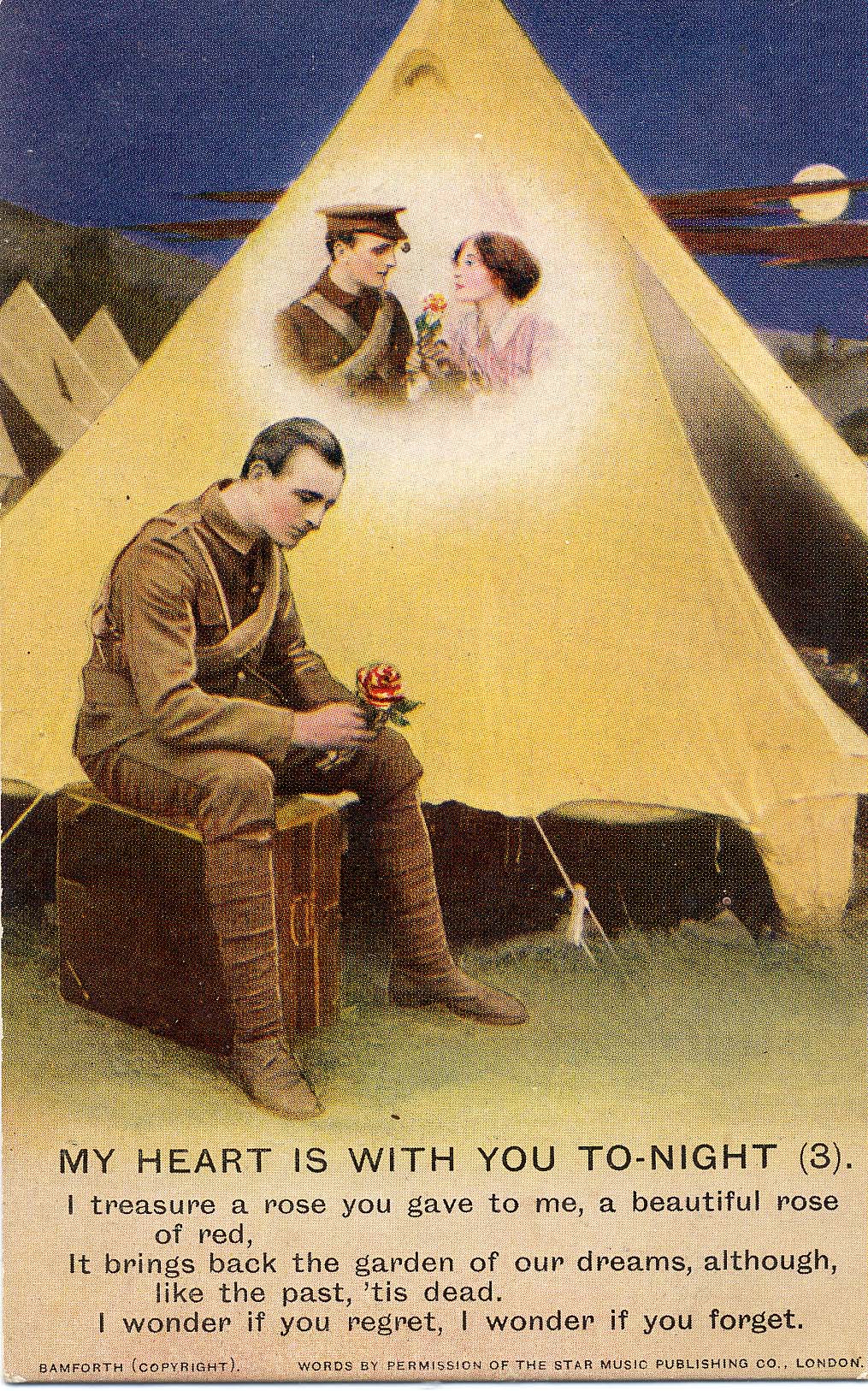The image is an artistic illustration that combines elements of a vintage photograph and digital enhancement. At the center sits a soldier dressed in a brown uniform, complete with a brown sash, brown pants, and brown shoes. He is seated on a brown suitcase or chest while holding a red flower with green leaves, gazing at it pensively. The background is dominated by a yellow tent set against a dark blue night sky, where a distant moon can be seen. There is grass on the ground beneath the soldier.

The tent features a thought bubble above the soldier's head, depicting a woman with short brown hair in a pink dress, indicating his contemplation of her. The poignant text at the bottom of the image reads:

“My heart is with you tonight.
I treasure a rose you gave to me,
A beautiful rose of red.
It brings back the garden of our dreams,
Although like the past, 'tis dead.
I wonder if you regret. I wonder if you forget.”

Additionally, a small copyright notice at the bottom reads "Bamforth Copyright Words by permission of Star Music Publishing Co-London."